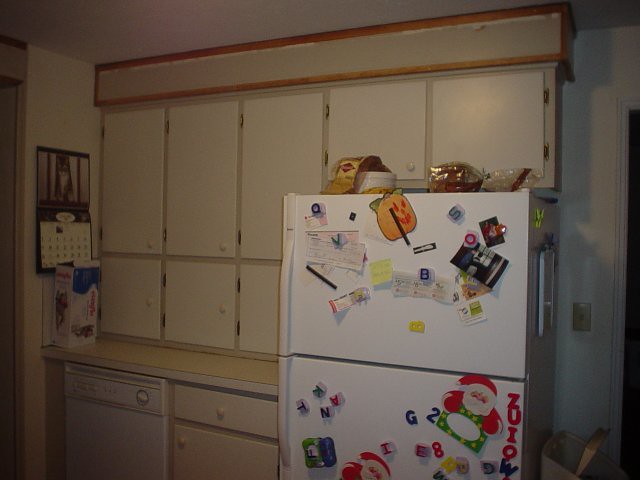This indoor color photograph captures a dimly lit kitchen featuring a predominantly white color scheme. The focal point of the image is a white refrigerator, positioned slightly lower and to the right of center, adorned with a myriad of magnets and notes. The lower section of the refrigerator, the main door, displays a Santa Claus magnet amidst a jumble of letters and kid-related items like random letters. The upper freezer section is cluttered with checks, coupons, and various notes, all held up by magnets. Surrounding the refrigerator are plain white rectangular cabinets with simple knobs, organized neatly above and around the fridge. To the left of the scene, a calendar is affixed to the wall, though its details are indiscernible. A white dishwasher is also visible beneath the countertop on the left side. The photograph, taken at a slight angle, suggests a living space designed with both adults and children in mind, as evidenced by the mixed assortment of items on the refrigerator. Despite the low light and a slightly out-of-focus capture, the scene reveals a cozy, lived-in kitchen atmosphere.